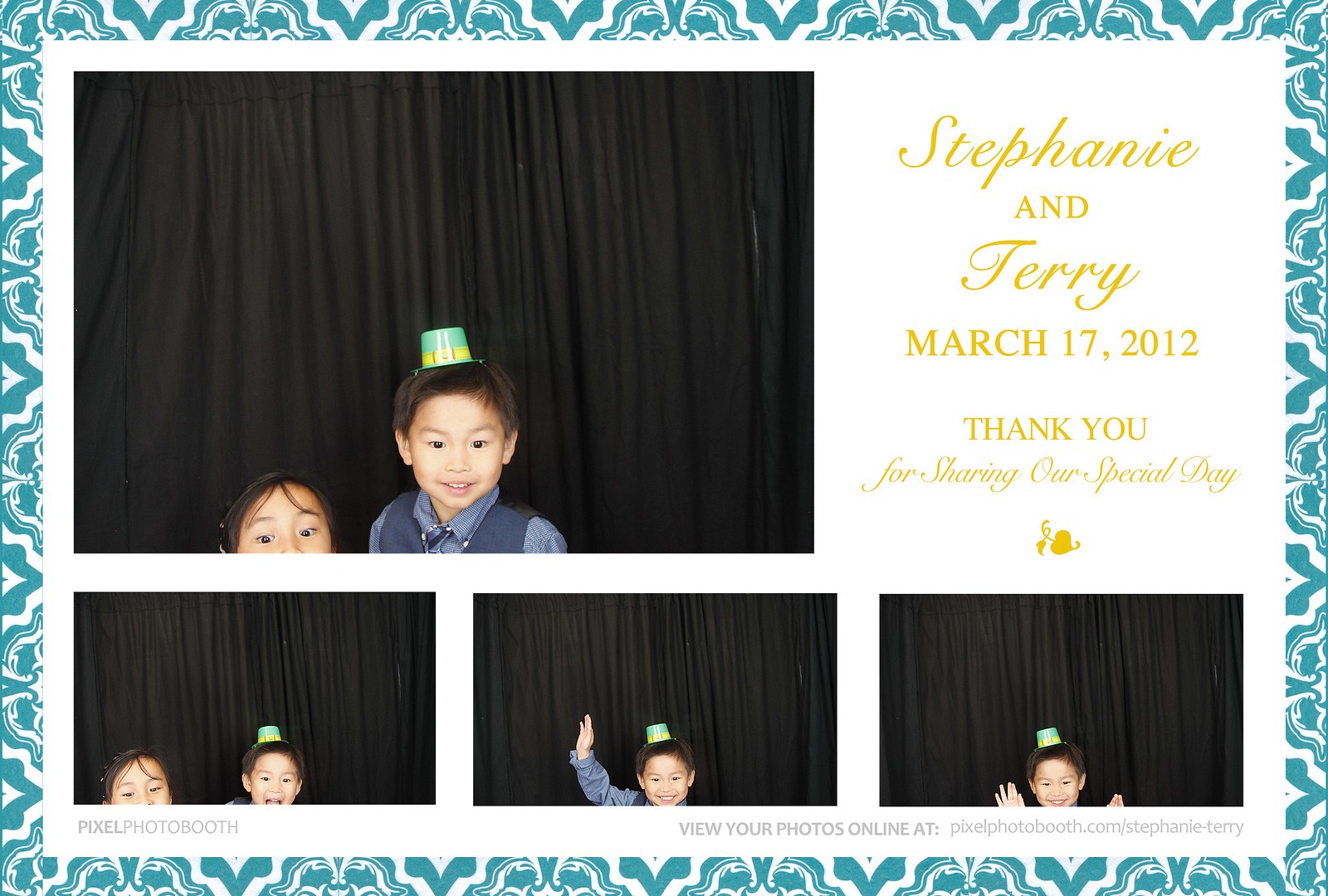The image is a thank-you promotional card with a clean white background, bordered by stylized turquoise shapes creating a decorative frame. The text in the center and top right corner is in cursive yellow font that reads "Stephanie and Terry, March 17th, 2012. Thank you for sharing our special day."

The card features four photographs: the larger one at the top left and three smaller ones along the bottom. The photographs predominantly feature two children. The larger top left photo includes a young boy with a beaming grin, wearing a green leprechaun hat and a button-up shirt, standing in front of a dark curtain. Beside him is part of a girl's face, seen only from the top of her nose up, with black hair. Among the three smaller photos at the bottom, two show the same boy, and the remaining one captures both children.

The card presents a cohesive feel with its blue and gold color palette, suggesting it might depict a playful moment taken from a photo booth at a wedding, celebrating Stephanie and Terry's special day. The bordered photographs have a distinct personal touch, thanks to the varying poses and expressions of the children, adding to the festive and appreciative tone of the card.